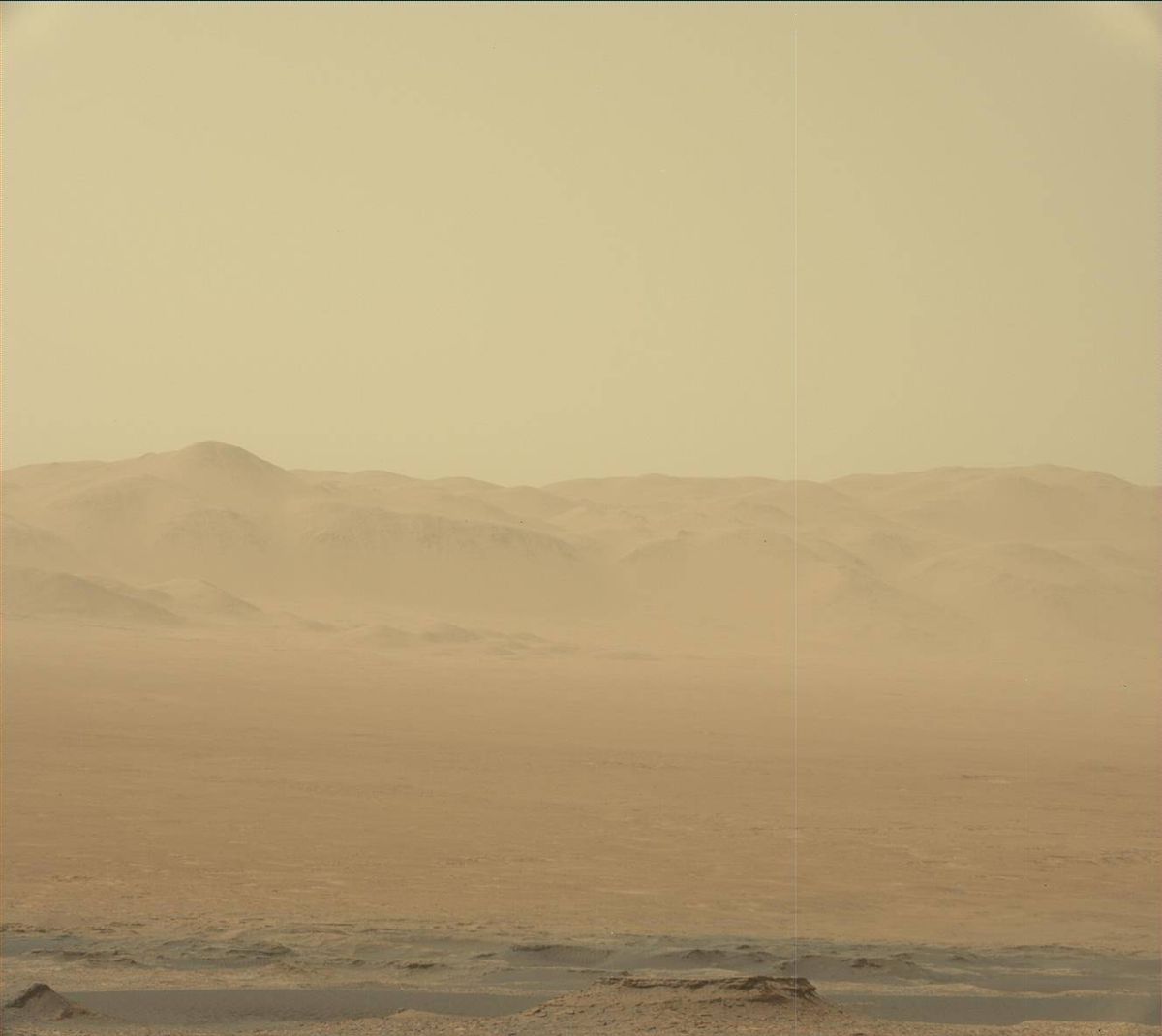The image depicts a vast desert landscape composed predominantly of dark brown sand stretching across a flat, expansive plane. The scene appears grainy and has a vintage, sepia-toned quality, giving it an aged and weathered look. The background features hilly formations or low sand dunes that add depth to the otherwise flat terrain. The sky blends seamlessly with the sandy ground in a lighter beige hue, likely due to a thick layer of dust or fog, reinforcing the image's overall hazy and indistinct appearance. The foreground displays a slightly darker, perhaps wetter, patch of sand or mud, providing the most clarity and contrast in the image. This combination of elements—grainy texture, muted colors, and indistinct features—creates a desolate and barren atmosphere.